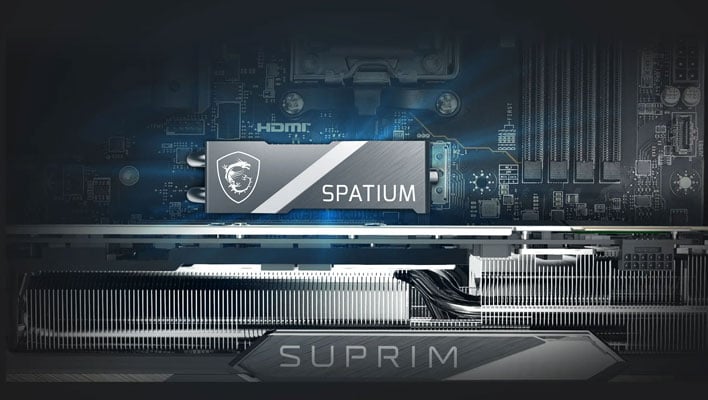The image depicts a detailed close-up of a computer motherboard, showcasing several technical elements. Central to the scene is a black, gunmetal grey block etched with the name "Spatium" (S-P-A-T-I-U-M) and featuring a shield insignia with a serpent or dragon-like creature inside. This block appears to be an integral part of the motherboard, possibly representing a brand or product. Above this block, the text "HDMI" is visible, indicating the presence of an HDMI connector, suggesting its use for connecting a computer screen or high-definition TV. The motherboard's surface displays intricate circuit patterns, wires, and components typical of advanced electronic devices. At the bottom of the image, in a similar grey etched style, the word "Suprim" (S-U-P-R-I-M) is inscribed, likely denoting another product or model associated with the primary brand "Spatium." The overall aesthetic emphasizes high-tech design and precision engineering within the realm of computer hardware.